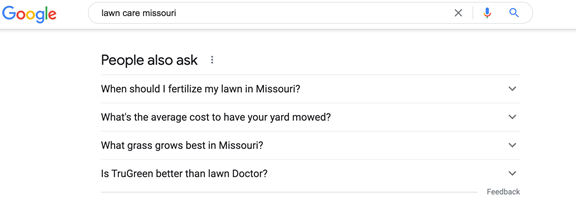A screenshot of a Google search inquiry prominently displays the Google logo in the upper left-hand corner. The logo features a capital G in blue, followed by lower-case letters: a red O, a yellow O, a blue G, a green L, and a red E. The search bar contains the query "lawn care missouri" in all lower-case letters. At the end of the search bar, icons for an X, a microphone, and a magnifying glass are visible. Below the search bar, it says "People also ask" with a list of recommended queries: "When should I fertilize my lawn in Missouri?", "What's the average cost to have your yard mowed?", "What grass grows best in Missouri?", and "Is TruGreen better than Lawn Doctor?". Each query has a drop-down menu to access additional information. There is also a link for providing feedback on the inquiry. The majority of the screen has a white background.